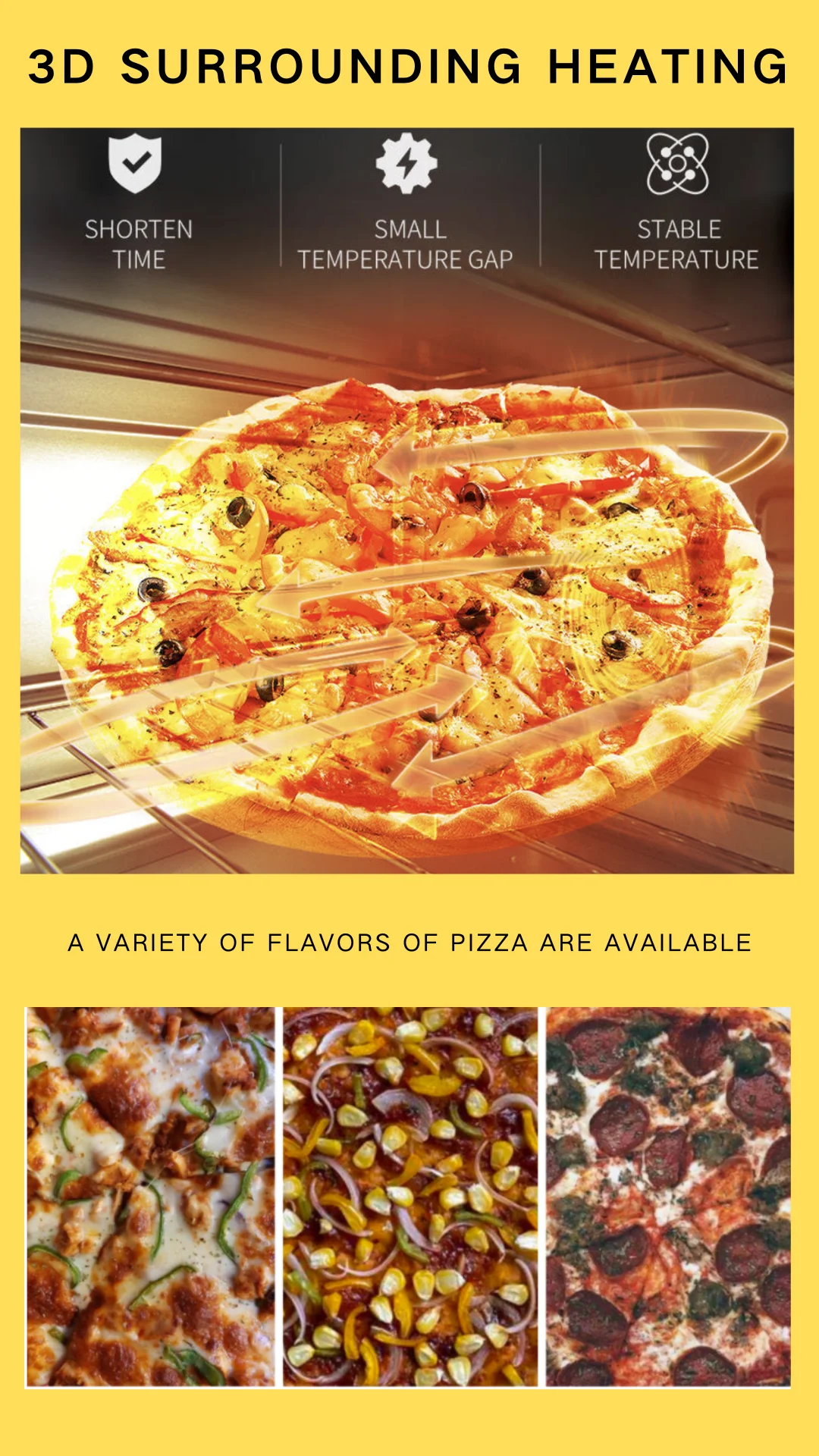The image features a diverse selection of gourmet pizzas, each showcasing unique toppings and ingredients. At the center, there's a schematic representation of a heating mechanism, depicted with gears and a lightning bolt, symbolizing stable temperature regulation. Around this, atoms and nuclei are artistically illustrated, emphasizing the precision of the cooking process. One pizza is adorned with a vibrant combination of melted cheese, slightly charred to perfection, alongside red sauce. Another highlights white cheese, brown meat, and green sliced vegetables, offering a variety of flavors. There's also a creative pizza topped with peanuts and onions, and another featuring black pepperonis and black sausages, contrasting with the red and white cheese, illustrating the innovative ingredient combinations available.